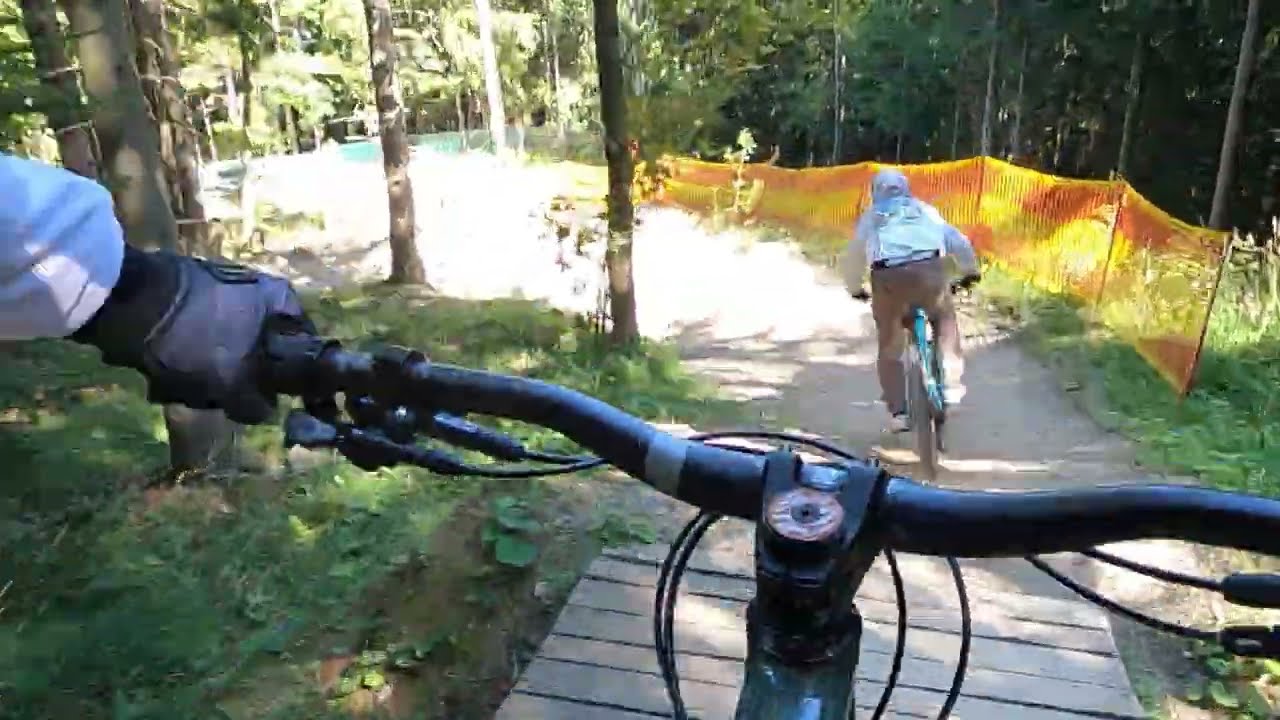The image depicts the perspective of a biker on a race track, captured as if the viewer is seated on the bike. In the foreground, black handlebars with visible brakes are gripped by a gloved hand. The biker is navigating a wooden bridge portion of the trail, surrounded by lush outdoor scenery. Ahead, another racer, identified by their tan pants, white sweatshirt, and helmet, rides a turquoise bike. The track curves to the left and is lined with an orange and yellow portable fence designed to keep bikers on the path. The path is well-lit by the sun, making detailed examination difficult, but it appears to be a mix of dirt and grass. The background features a dense array of trees, grass, bushes, and additional greenery, all characteristic of a natural park setting. The image captures the thrill and environment of a mass mountain biking trail.